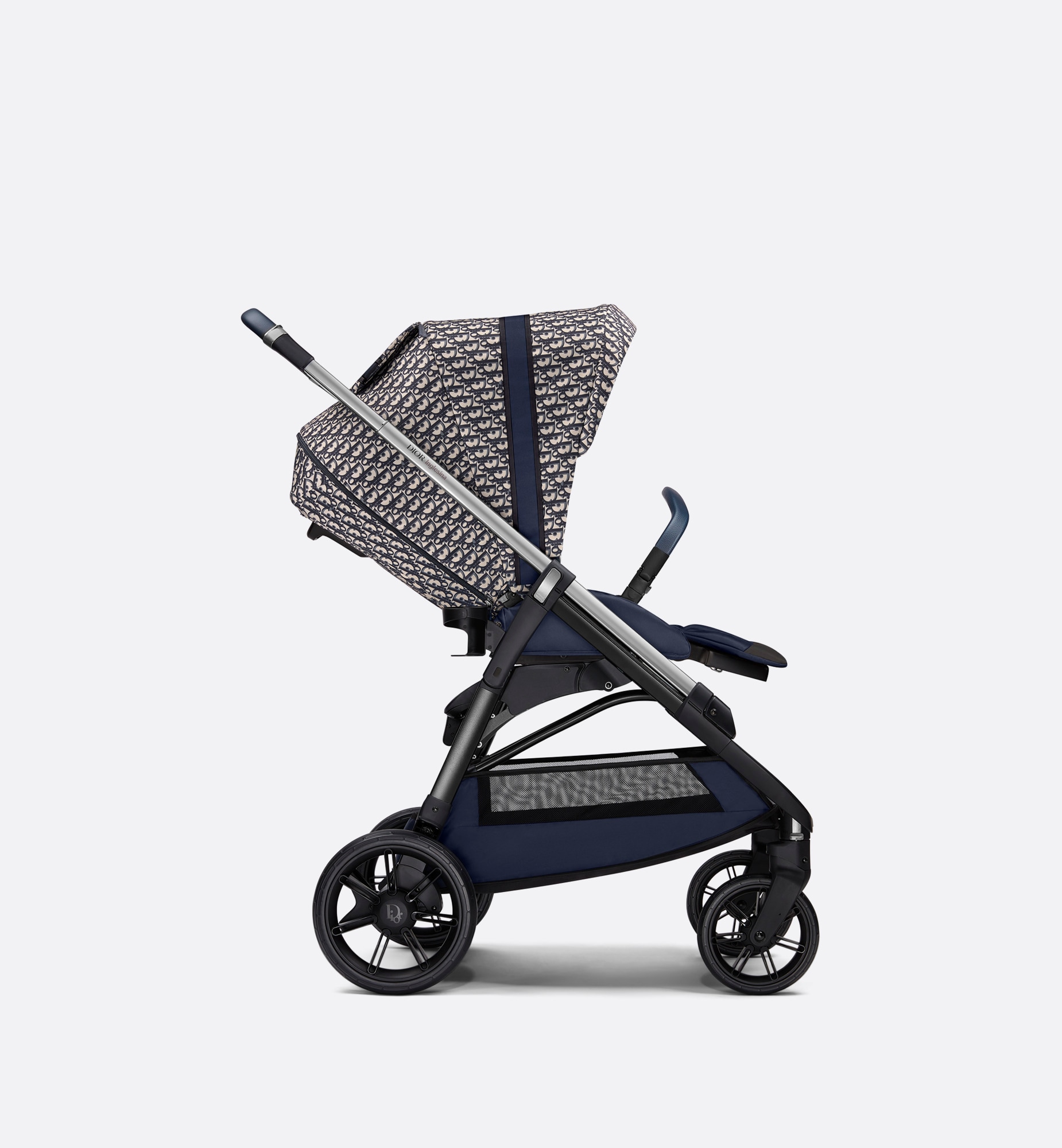This detailed photograph showcases a modern infant stroller set against an off-white background. The stroller sits on a white floor and is surrounded by white walls, creating a stark contrast with its predominantly dark blue and black design. The stroller features four black wheels, with the rear wheels being notably larger than the front ones, which are designed to pivot for easy maneuverability. 

The base of the stroller, which includes a storage space made of dark blue fabric with black mesh sides, is supported by silver, aluminum, metallic support brackets and bars that extend upwards and form the handle. The handle grip itself appears to be either black or dark blue. 

The stroller is equipped with a large canopy, primarily monotone black and off-white with a distinct dark blue band running across the top. The canopy, which is adorned with a subtle gray design that resembles tiny heads, provides ample coverage for the infant. The interior of the stroller, including the seat and its safety belt, is dark blue. Notably, the design of the stroller allows for the possibility of removing the seat with the canopy to serve as a car seat, showcasing its versatility and unique, modern design.